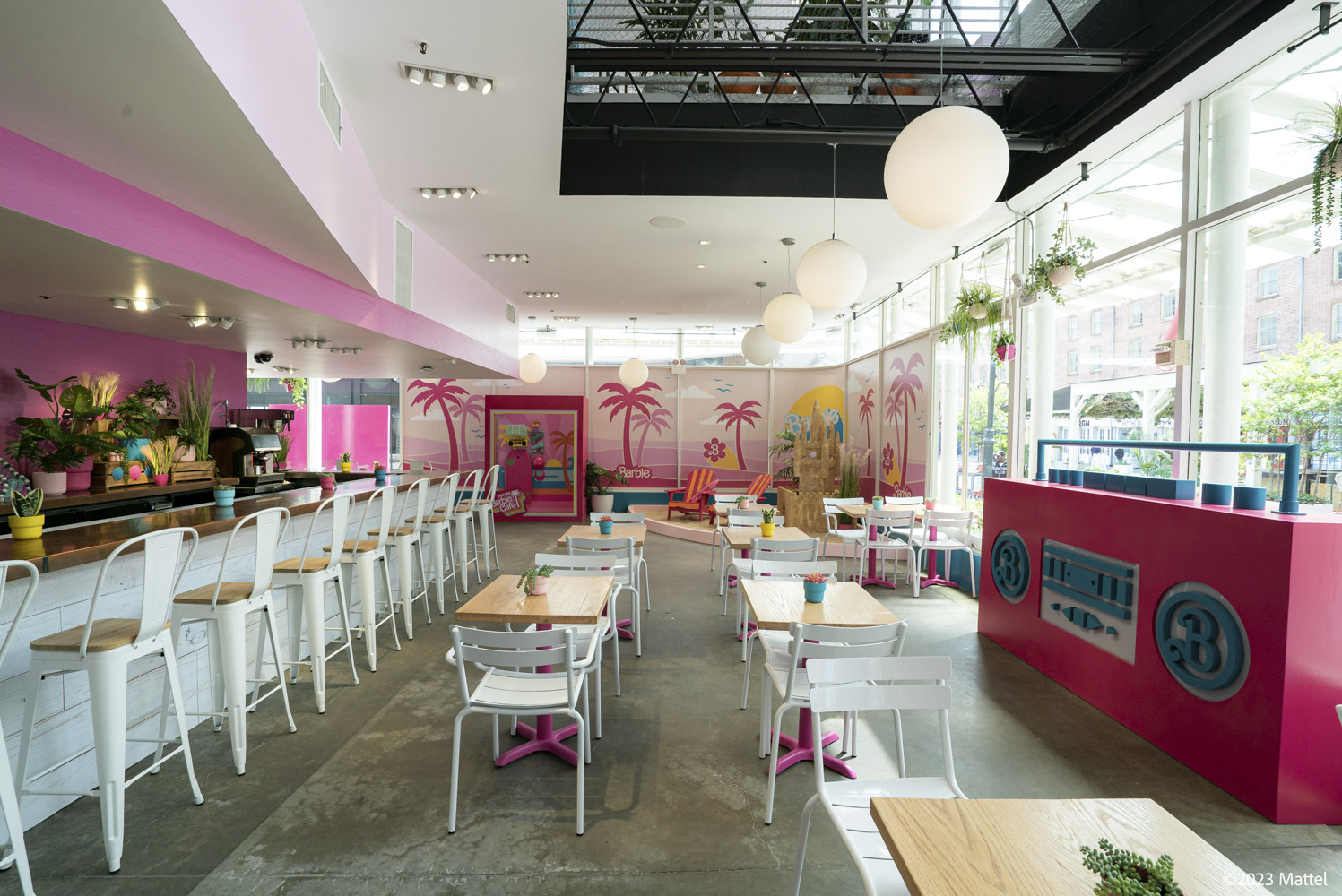The photograph captures the vibrant interior of a Barbie-themed cafe. On the left side, there's a long bar top with numerous white stools with wooden seats lined up against it. Above the bar, a glossy pink strip adorns the wall, enhancing the aesthetic along with various potted plants in colorful pots. Behind the bar and extending into the center of the room are small tables, each capable of seating two people, with hot pink stands and small potted plants on top.

The right side of the image is dominated by large windows that let in ample natural light, making the space bright and welcoming. In front of these windows, there is an enormous pink boom box, whimsically designed as an art piece with "B for Barbie" displayed prominently on the speakers. This boom box adds an element of playful decor that harmonizes with the overall Barbie theme.

In the background, a charming beach scene unfolds with a sandcastle prop and walls painted with pink palm trees, further cementing the vibrant, playful atmosphere. The white ceiling is dotted with globe lights and directed spotlights, ensuring the entire area is well-lit. The cafe’s distinct color palette predominantly features bright pink and white, giving it a cheerful and fun vibe reminiscent of a Barbie dream world.